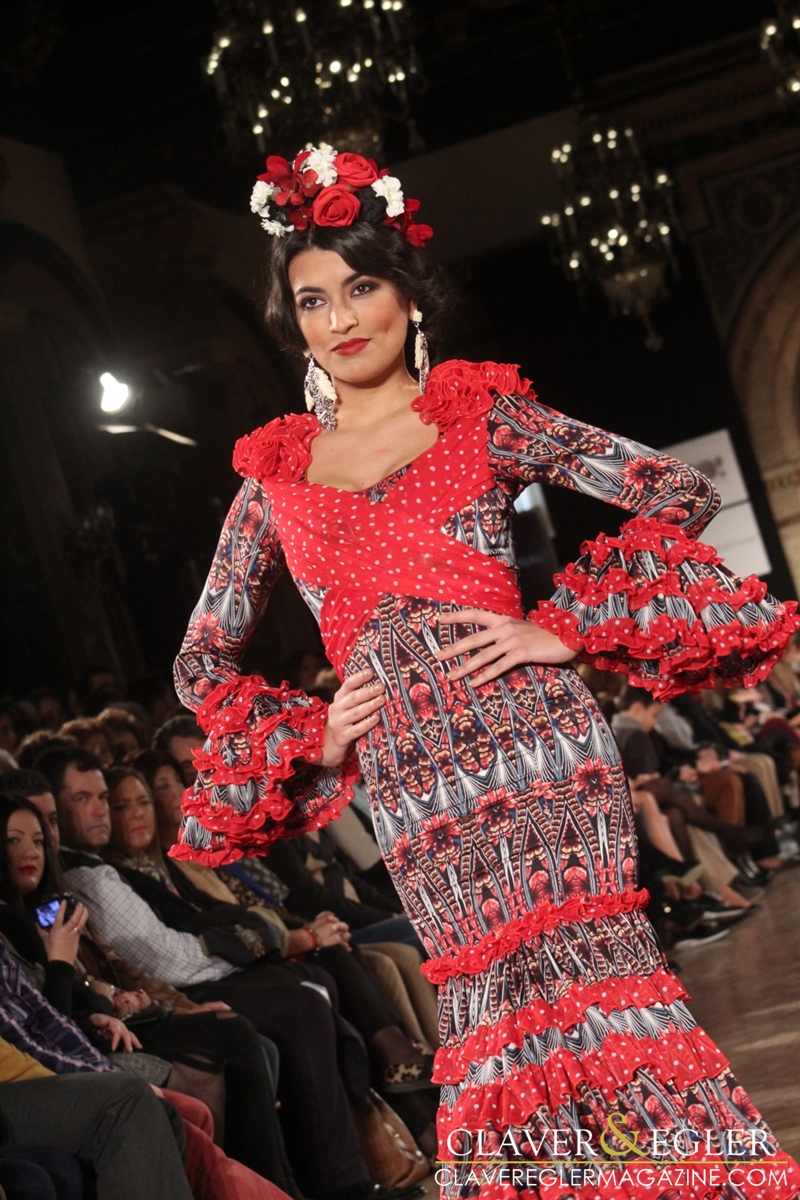In this richly detailed image, a tan-skinned model with dark black hair is confidently striding down a runway with her hands firmly placed on her hips. She sports a unique, eye-catching dress primarily in red, accentuated with gray, white, and dark purple hues. Her ensemble is highly ornate, featuring complex patterns and textures; the upper chest showcases a red crisscross design with white dots, while the shoulders are adorned with fluffy red flowers. The sleeves transition in color and material from red, white, and purple down to wide, encircling bands of red, black, and white at the wrists. Her lower dress features intricate red and white circular patterns and encircling strips that cascade down her legs, concealing her shoes. 

Her fierce, determined expression is highlighted by red lipstick, large, feathery white, and grayish earrings, and a dramatic bouquet of red and white roses pinned to her hair. A vibrant assortment of lights illuminates the scene from the ceiling, adding to the elegance and grandeur of the setting, which is atmospherically enhanced by chandeliers in the background. Seated spectators line the left side of the runway, their attention fixated on the model’s striking appearance and commanding posture. This high-fashion event takes place in a clearly upscale location, emphasizing the sophisticated ambiance. In the lower right corner of the image, the text "Claver & Eggler" alongside the website "ClaverEgglerMagazine.com" indicates the prestigious publication capturing this memorable moment.